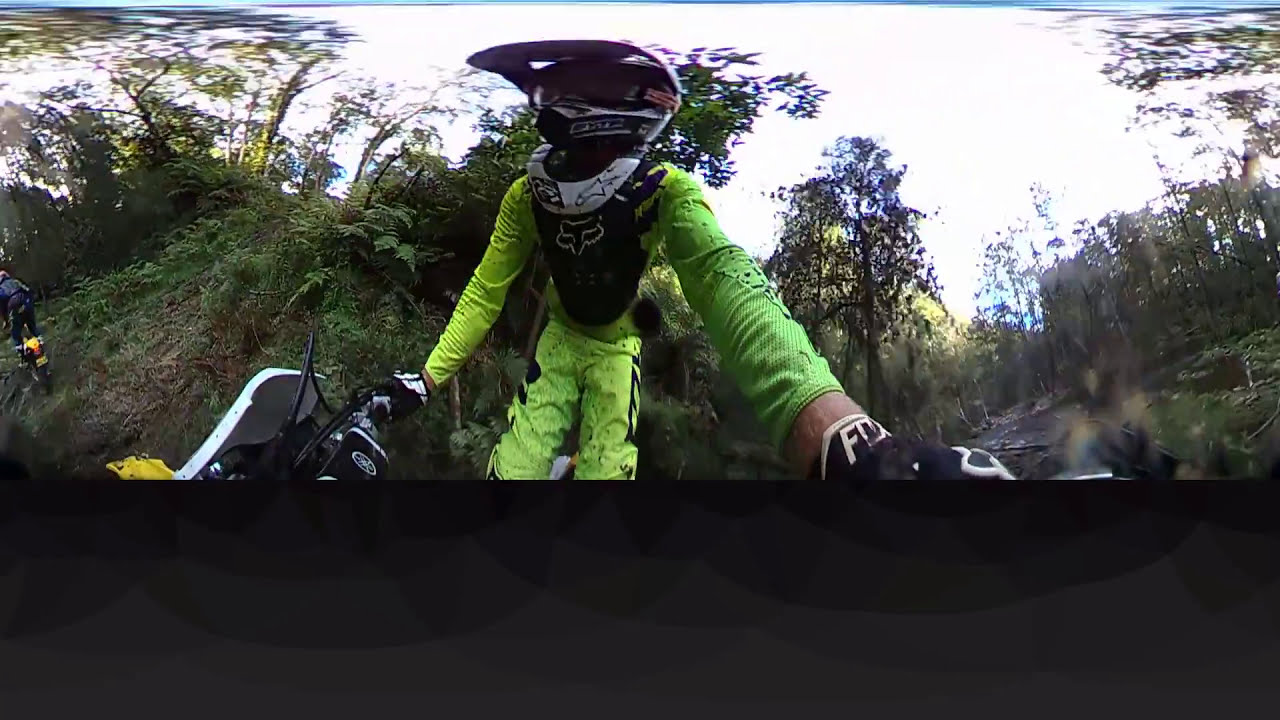In this dynamic image, a central figure dominates the scene, a man attired in complete dirt biking gear, including a black and white helmet, eye goggles, a lime green long-sleeved shirt, matching pants, and black gloves. His torso appears black, possibly due to either padding or the design of his shirt. Riding a dirt bike through a verdant forest, the camera, seemingly mounted on the handlebars, captures the rider's forward-facing perspective, creating a slightly distorted and fisheye lens effect, with notable warping and blurring at the edges. The scene is bustling with greenery; various trees, bushes, and brush envelop the rider, suggesting a thickly wooded outdoor setting. Light filters through, indicating a cloudy yet bright midday. To the left, partially obscured by the vegetation, another dirt bike is faintly visible, hinting at a fellow rider either ahead or behind. The terrain suggests a rugged trail, possibly sloping from a hill or mountain, with what appears to be a river or water feature splashing up in the background, adding to the energetic and adventurous atmosphere of the image. No textual elements distract from the immersive outdoor experience captured here.